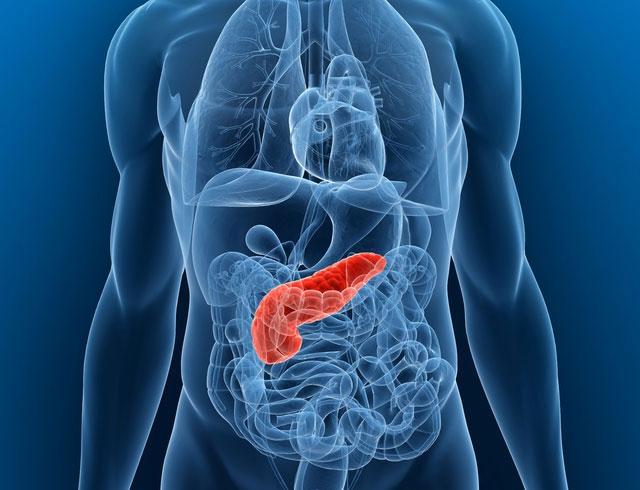The image is a highly detailed scientific diagram depicting the anatomy of a human male body. The entire diagram, including the background, is rendered in various shades of blue, with a deep navy blue serving as the backdrop. The translucent body in the center allows for a clear view of the internal organs, which are also shown in blue. These include the lungs, heart, stomach, intestines, kidneys, liver, pancreas, and gallbladder. The torso and arms are visible, but no bones are shown, focusing solely on the organ systems. In the central area, around the upper abdomen, one particular organ is highlighted in red, contrasting starkly with the otherwise blue palette. This red-highlighted region is situated near the intestines and is somewhat gun-shaped, though its exact identity isn’t labeled or immediately clear. This red highlighting draws attention to a potentially significant anatomical feature or focal point for further study.